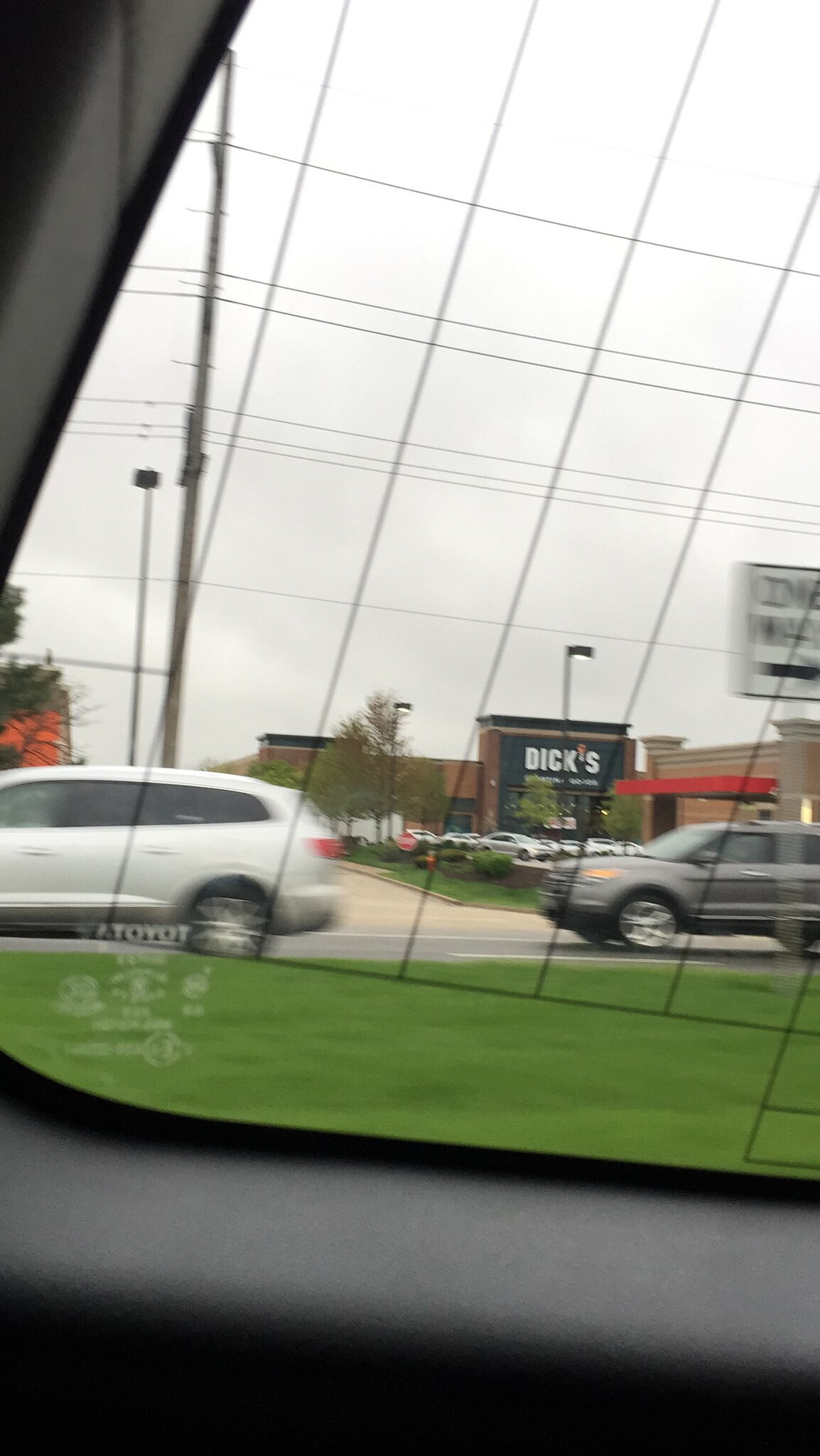This photograph captures a view from inside a moving vehicle, likely taken through either the side or rear window. The immediate foreground includes part of the vehicle's black plastic interior, positioned just beneath the window. The window itself is equipped with black defroster lines, which create a subtle grid across the glass.

Beyond the window, a strip of vibrant green grass separates the vehicle from a busy road where several cars are traveling in the opposite direction. The cars appear slightly blurred due to their motion, suggesting that the vehicle from which the photo was taken is also in motion. The sky above is overcast, casting a muted light over the scene, hinting that it may be close to sunset or possibly raining, although there's no direct evidence of precipitation.

In the distance, a shopping area comes into view, with the most prominent sign reading "Dick's Sporting Goods," indicating the presence of a retail complex. Notably, the street lights remain off, adding to the overall dim and subdued atmosphere of the photograph.